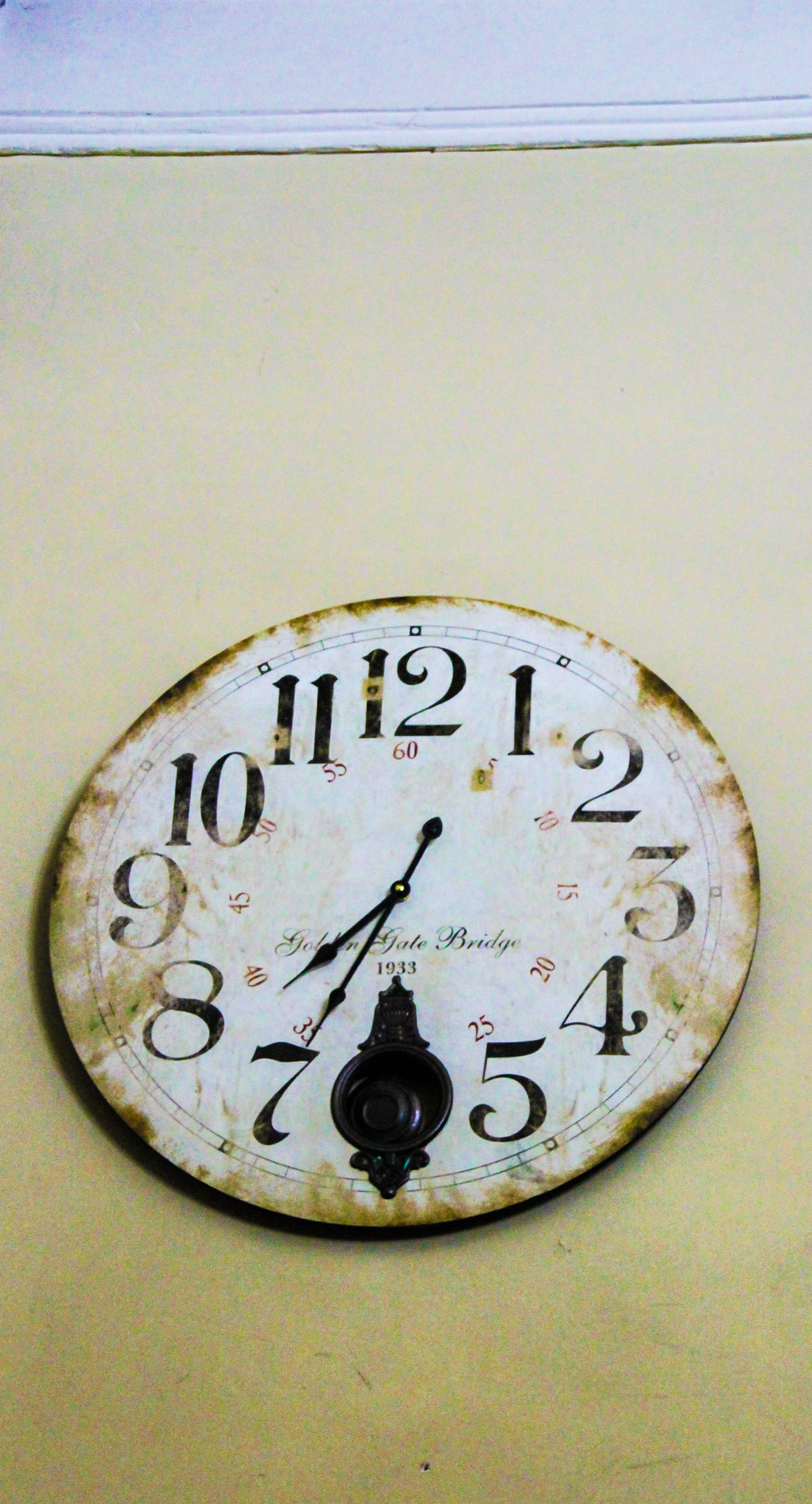This image features a distinctly vintage-style wall clock, prominently displaying only its face plate without any encompassing bezel or frame. The clock emanates an aged aesthetic, characterized by a deliberately stained and worn exterior edge, though it remains uncertain whether this wear is authentic or artificially created to mimic antiquity. This ambiguity extends to the potential presence of a modern mechanism within the clock, suggested by the relatively pristine condition of the minute and hour hands.

The clock face, predominantly white beneath the intentional smudging, is adorned with the full sequence of twelve Arabic numerals encircling its analog display. Notably, at the position traditionally occupied by the numeral six, there is an emblematic logo, above which the year "1933" is inscribed—a detail uncommon among vintage timepieces, thereby hinting at the possibility of it being a reproduction. The setting for this captured image is a light tan or light brown surface, enhancing the contrast with the clock’s design and further highlighting its unique features.